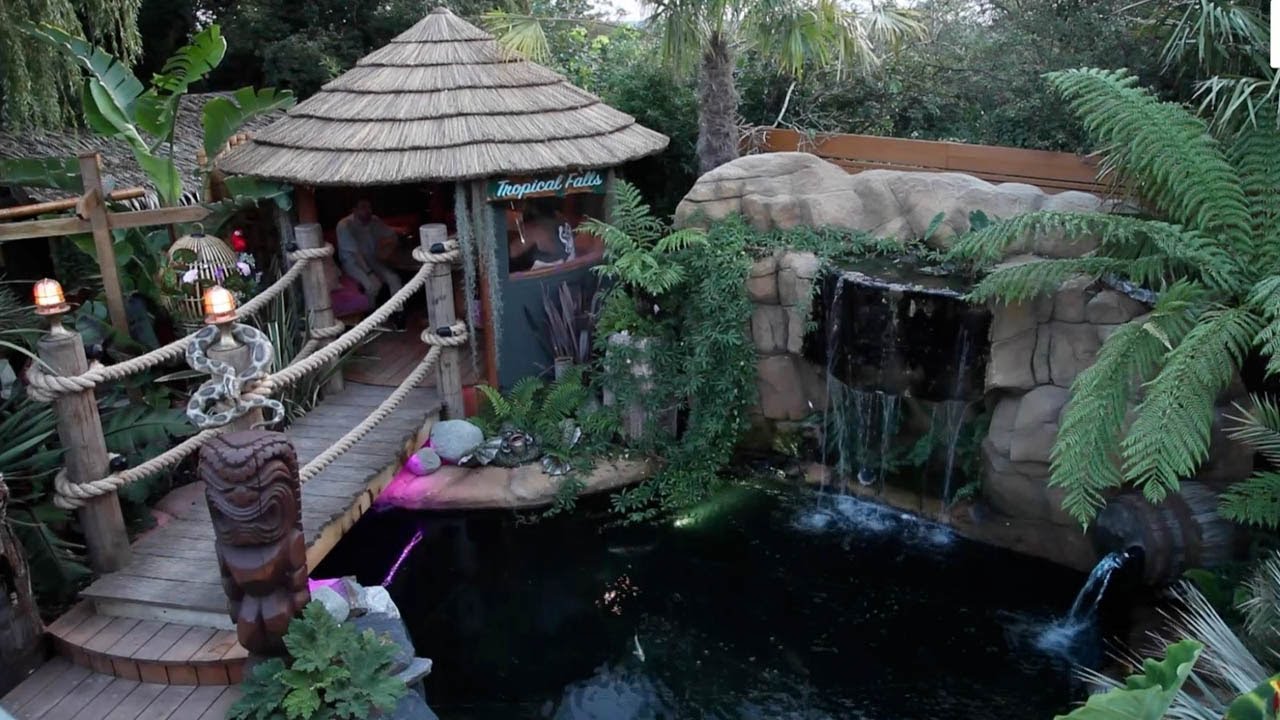In this high-angle shot, likely taken from a balcony, we're looking down at a tropical or tiki-themed setting, possibly within a theme park. Directly below us, there's a man-made lagoon with a few submerged lights. A rock wall above the lagoon features a cascading waterfall, which adds a serene touch as water pours into the lagoon. The rock wall is adorned with lush ferns and vines, enhancing the tropical feel.

To the left, a wooden tiki statue made of dark wood stands on a wooden bridge that spans the lagoon. This bridge is equipped with large rope guardrails, and a small snake statue with an attached lamp sits on one of these guardrails, adding to the theme. Nearby, there's a "Tropical Falls" sign, suggesting a possible name for this area. 

Adjacent to the bridge, there's a grass-roofed hut or gazebo where people are seated around tables, indicating an eating area. This space looks inviting and vibrant, complementing the overall theme with its natural and constructed elements harmonizing together.